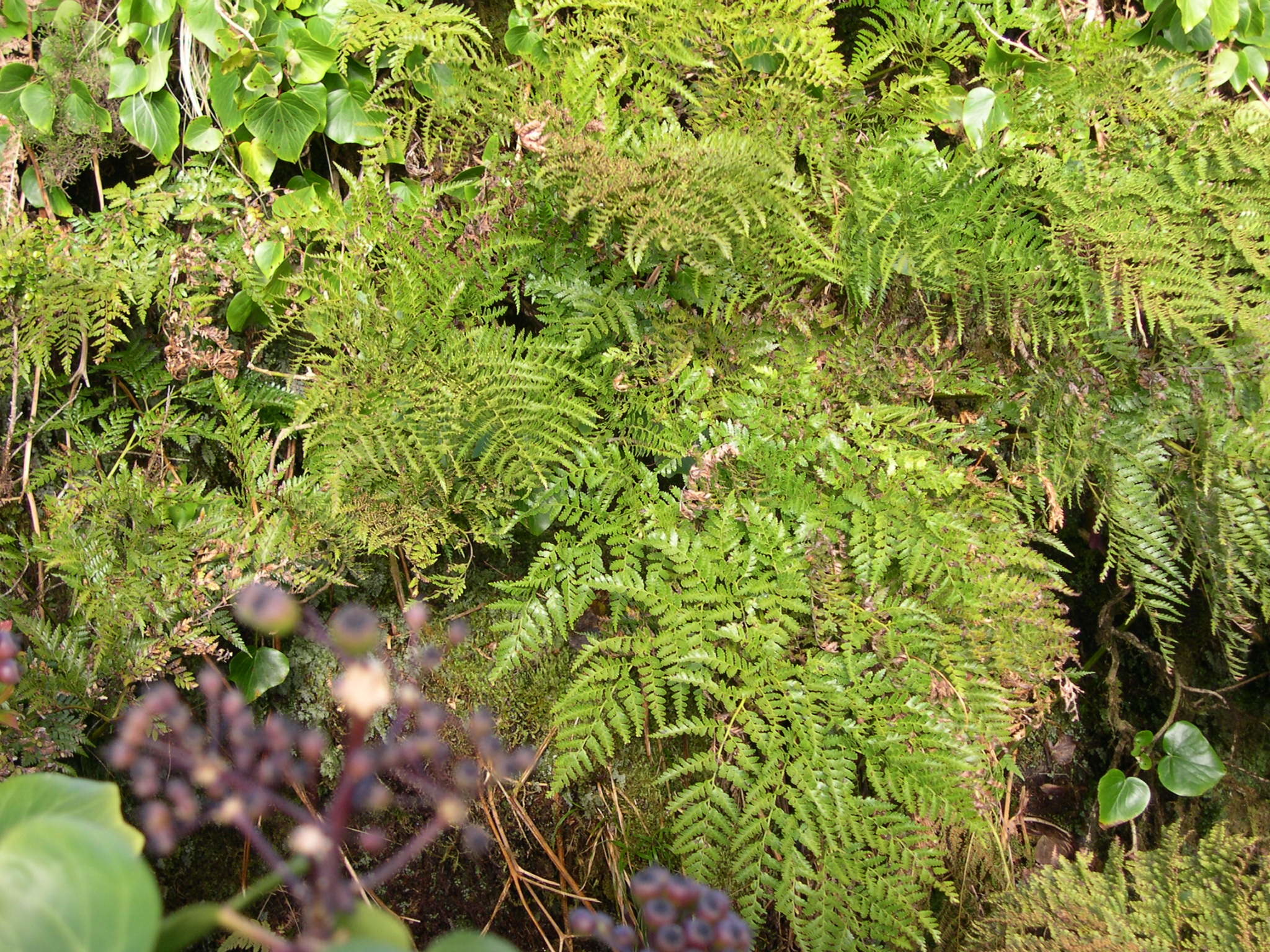This outdoor daytime image features vibrant plant life with various green and leafy elements. Dominating the center are lush, green ferns with long stems extending to triangular tips, showcasing leaves that widen toward the plant's base. Toward the lower left-hand corner, a purple-stemmed plant with dark, almost black buds is visible but out of focus, surrounded by green leaves. Additionally, the bottom right corner reveals two or three heart-shaped leaves, shiny and healthy, echoing similar foliage at the image's top left. The ferns, appearing to grow on or around a rocky hill, showcase a rich display of nature's intricate details and textures.